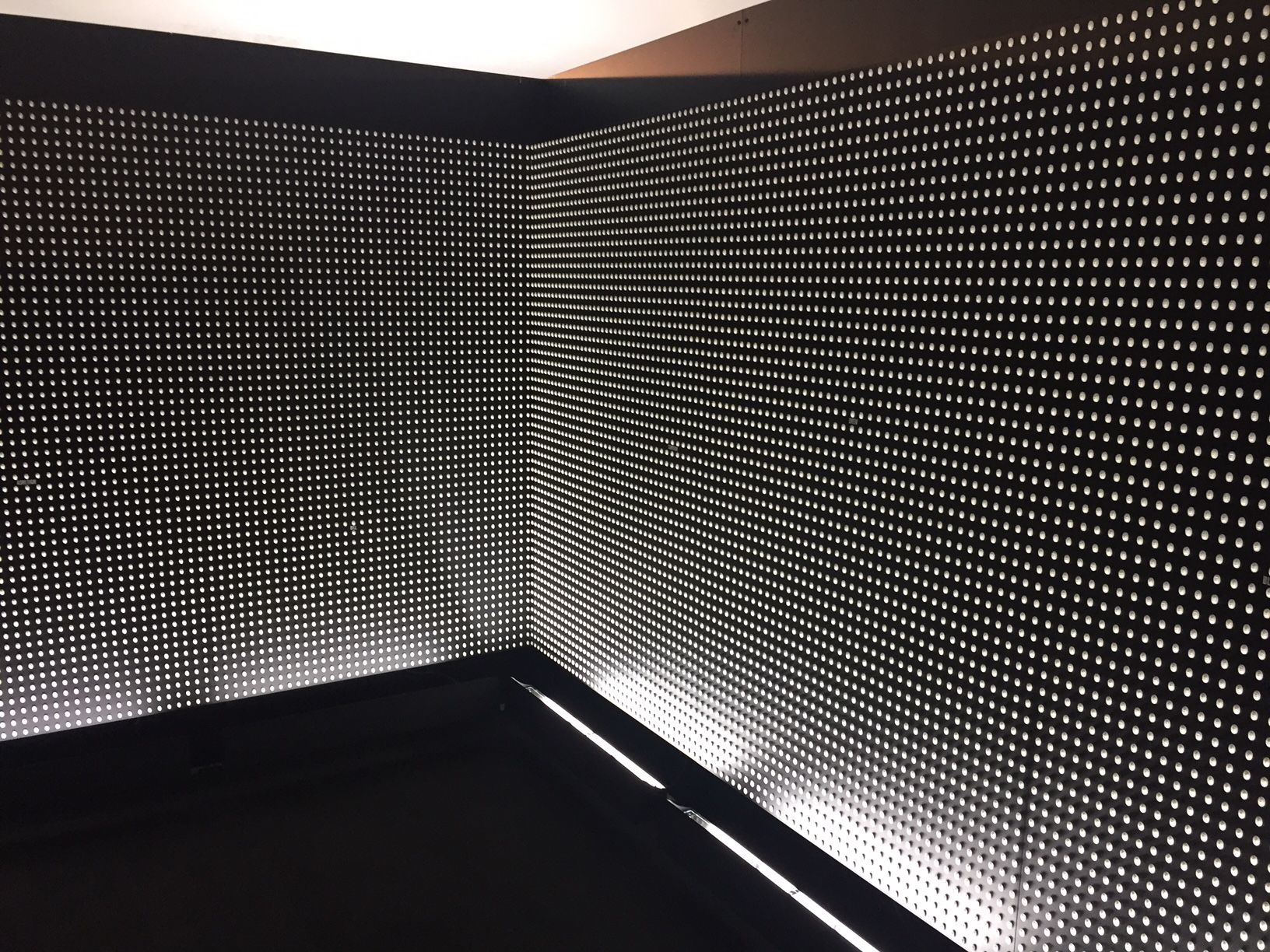The image depicts an abstract corner scene that could be interpreted as either part of a box or a room. The composition features two black walls adorned with a grid of small white dots, which might be tiny embedded lights or protrusions. These dotted walls are lit from below by strip lighting, illuminating the bottom portions. The corner of these walls converges slightly to the left of the image's center, with a black floor visible along the bottom left and middle. Above the black walls, a transition occurs where the top area is light in color, indicating a ceiling. To the right, a brown element suggests either a wall or ceiling, contrasting with the overall monochromatic theme.